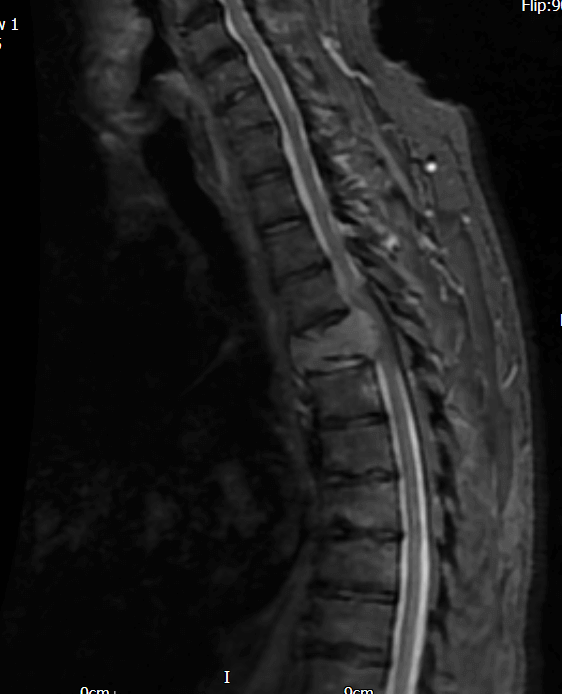The image is a black and white, vertically rectangular x-ray depicting a detailed view of a spine against a black background. Positioned centrally, the spine is displayed with a slight vertical curve. You can clearly observe the vertebrae, discernible as individual bone structures, with the intervertebral discs appearing as horizontal lines between them. The spinal cord, trimmed in white with a darker interior, is visible running through the vertebrae. Notably, there is an area where the spinal cord appears to project outward, possibly indicating a rupture.

Text in white appears in several places: at the top left, it reads "FLIP: 9 1", and at the bottom left corner, it says "OCM". Additionally, there are markings denoting measurements – "0 cm" appears twice, once in the middle and once further to the right. The left side of the image is labeled with a tiny "V1". The image also depicts surrounding anatomical structures, likely cartilage and skin, on the right side of the spine. Overall, this is a high-resolution x-ray focusing intricately on the spine and its immediate vicinity, highlighting both the internal and external anatomical features.